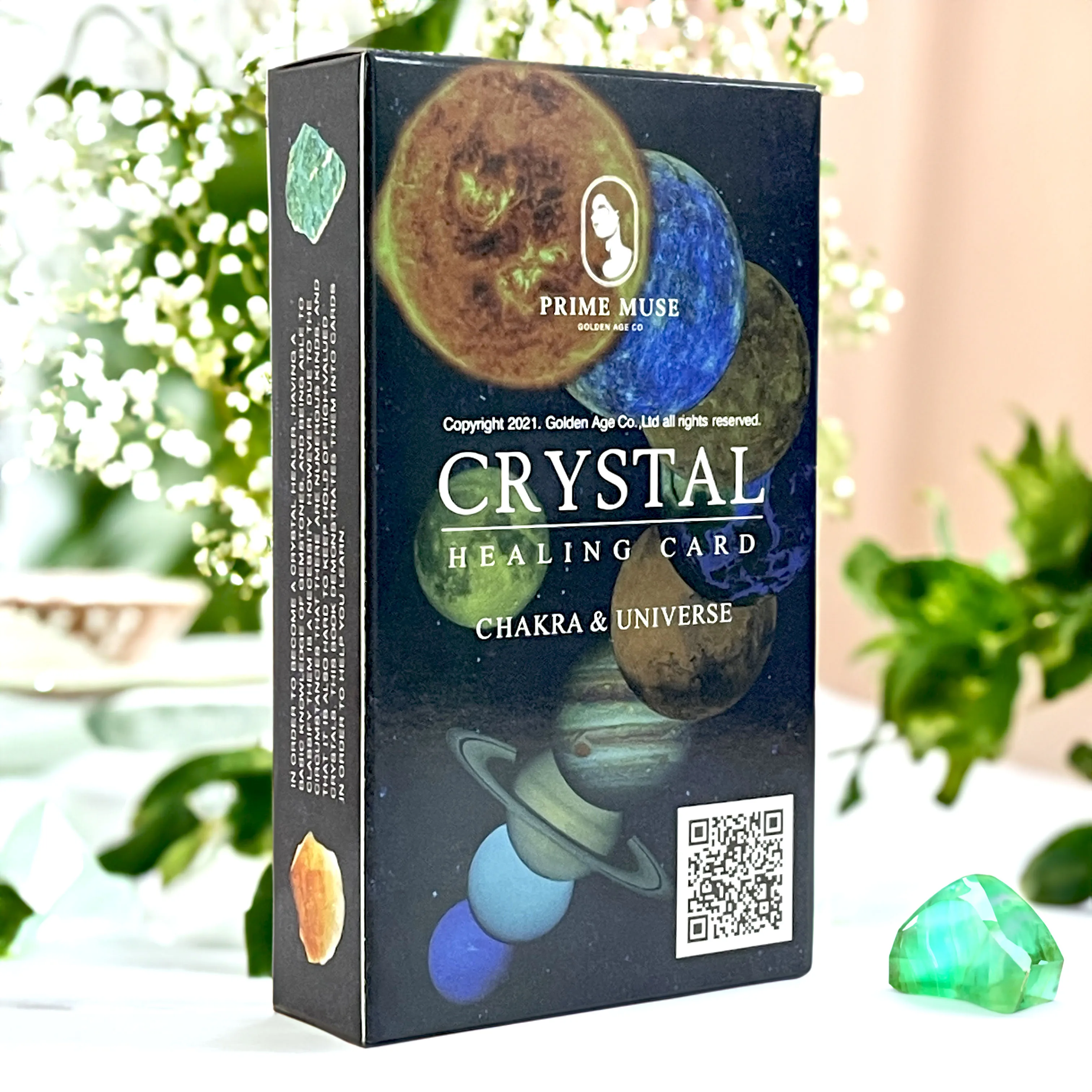This color photograph features a rectangular black box that extends from the top to the bottom of the image, labeled as "Crystal Healing Card" with the subtitle "Chakra and Universe". The box, a product of Golden Age Co. (copyright 2021), showcases an array of planetary illustrations cascading down the front side, including a glowing orange planet at the top, adjacent to a blue planet, and further below, an olive green, a purple-black, and other celestial bodies, ultimately leading down to a green planet in the center. The box also displays a logo with a woman’s face and "Prime Use, Golden Age Company" inscribed above the text. Additional information is printed vertically on the left side, featuring images of crystals. A UPC symbol is located at the lower right corner. The background reveals the box resting on a white table, accompanied by a green crystal to the right and some house plants, one with white flowers. A pink wall is slightly visible in the backdrop.